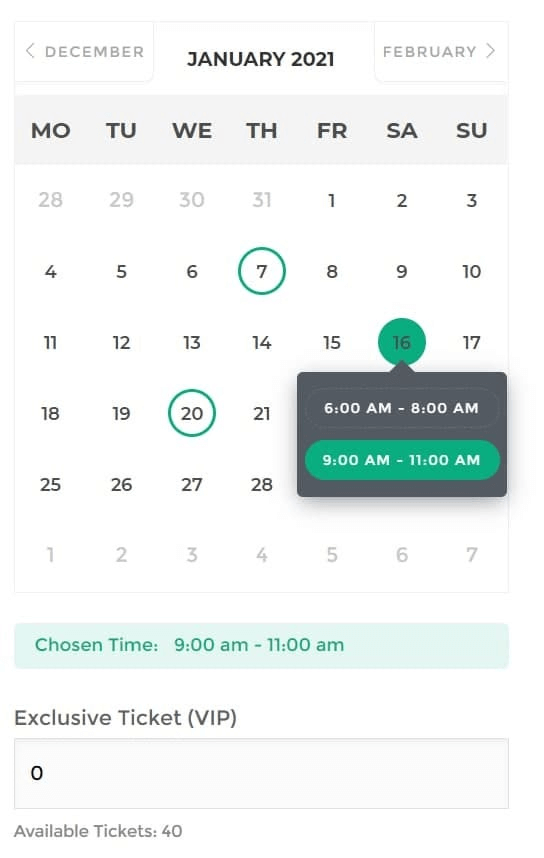The image depicts a map overlay on a calendar for January 2021, presented horizontally from Monday to Sunday. The dates are clearly marked until the end of the month. Notably, the 7th and 20th are encircled in green, suggesting their importance. The 16th is also encircled but has a filled green circle, indicating a special event. A grey annotation bubble points to the 16th, indicating two possible time slots: 6 AM to 8 AM and 9 AM to 11 AM, with the latter highlighted in green, indicating its relevance. Below this, a light green panel with darker green text confirms the chosen time as 9 AM to 11 AM. A section titled "Exclusive Ticket VIP" includes an input box with the default value of zero underneath. Further down, another section labeled "Available Tickets" states there are 40 tickets remaining.